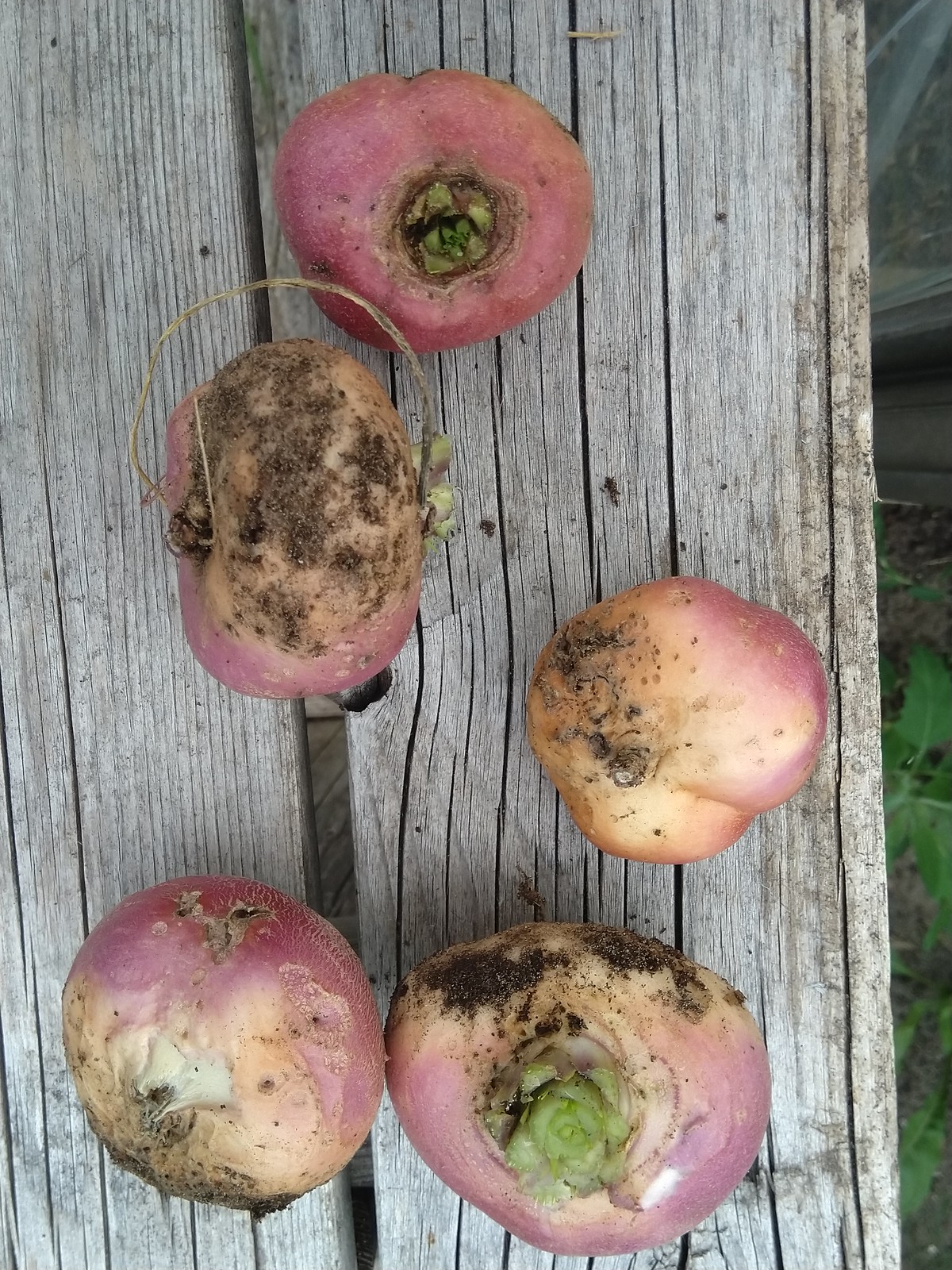In this detailed photograph, five purplish-skinned vegetables are displayed on a raw, weathered wooden surface that appears to be part of a deteriorating picnic table or wooden deck. The planks of wood, oriented vertically and showcasing prominent green and black weathering lines, highlight the rustic texture and age of the surface. The vegetables—though somewhat hard to distinguish—include red-skinned onions, red-skinned potatoes, and what seems to be a pomegranate. Each vegetable is covered with dirt and possesses varying shades of purple and red, with some showing green stems, eyes, or vines still attached. The placement of the vegetables is varied; one is almost standing on its side within a crack between two planks, while others lie upright or upside down, partially obscured by lingering roots. In the background, hints of ground vegetation like grass and weeds are visible, creating a natural, earthy setting.